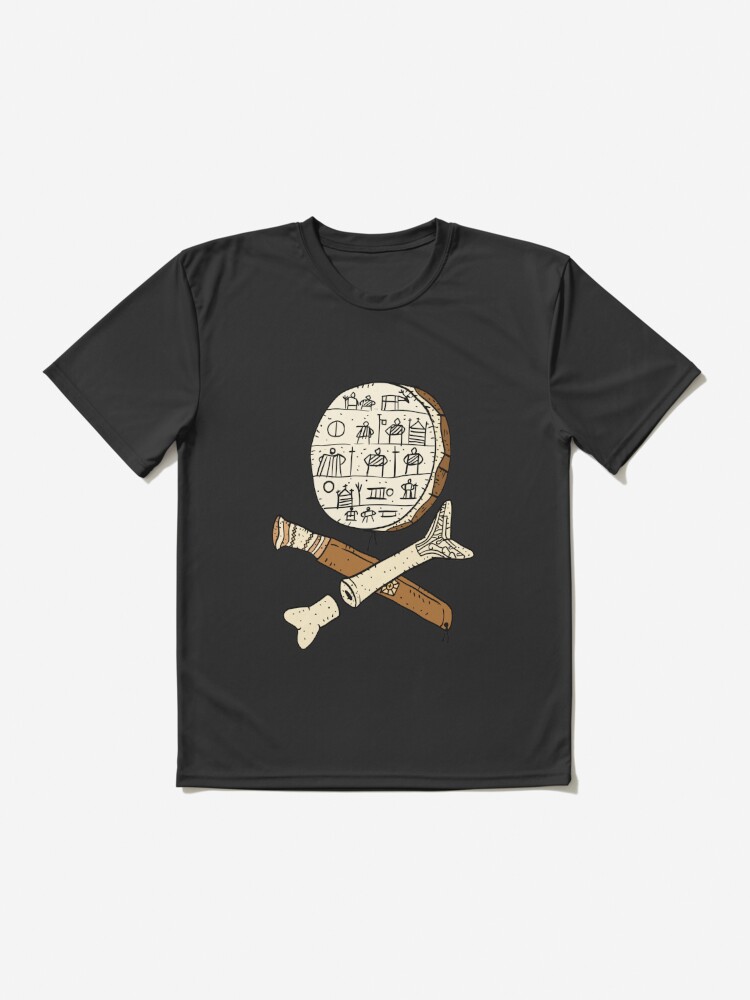In this image, a black t-shirt lies flat, revealing a striking and abstract graphic printed on its front. Central to the design is a white circle filled with doodle-like symbols, including stick figures, against a beige background. Beneath this circular emblem, there is a diagonal arrangement of objects: a broken fishbone-like figure in a beige-white hue crossing from bottom left to top right, and a brown club or bat with white tape on the handle extending from bottom right to top left. Together, these elements form an abstract crossbones motif. The entire design is rendered in shades of black, white, and brown, creating a visually intriguing and somewhat cryptic pattern that invites closer inspection.